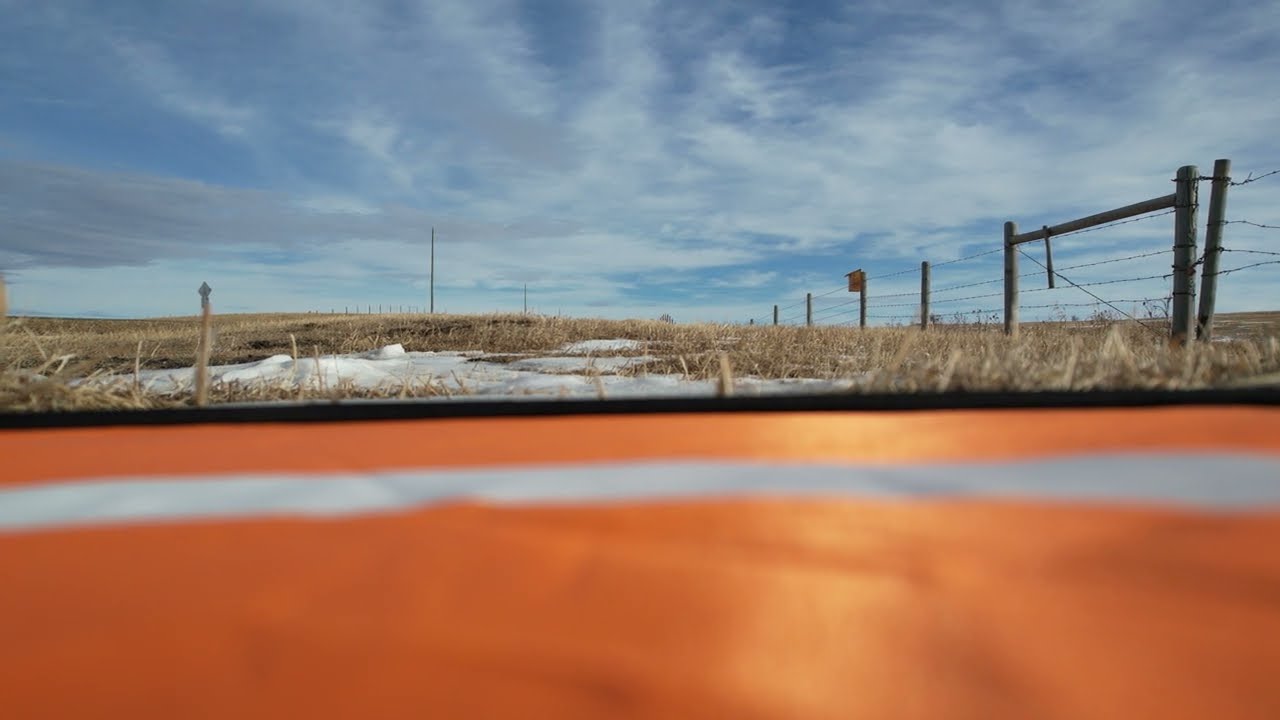In this horizontally rectangular photograph, an unusual ground-level perspective captures a multifaceted scene. Dominating the very foreground is a blurred, orange object with a white stripe running across it, possibly the top of a barrel or, more likely, a car hood upon which the camera might have been placed. Beyond this vivid foreground, the in-focus portion of the image features a field of dried, tan-colored grass interspersed with patches of snow. A barbed wire fence, supported by wooden posts, recedes into the distance. The serene backdrop includes a blue sky streaked with high, wispy clouds. Near the wiring, utility poles are faintly visible, adding to the scene's rustic charm. The overall ambience suggests a bright, outdoor daytime setting.